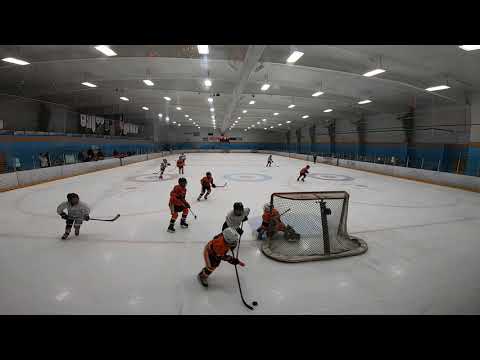The image depicts an expansive indoor ice skating rink where a youth hockey game is unfolding. From a vantage point behind the net, we see the goalie crouched in anticipation, dressed in an orange jersey and helmet. Likewise, an orange-clad player controls the puck behind the net, likely strategizing a move to outmaneuver the opponents and score. Players from both teams—one in orange, the other in white—are scattered across the rink, some advancing towards the puck handler.

The game's setting is well-lit by numerous fluorescent lights attached to the white ceiling, which is adorned with banners on the left side. The rink itself features blue and white walls with an orange stripe running horizontally along the middle. Central to the ice, large blue circles with orange centers mark important gameplay areas. Though there are some spectators in the stands, they are sparse, lending a sense of it possibly being a practice session rather than a full-scale game. The size of the rink is notably large, emphasizing the arena's grandeur despite the few attendees.